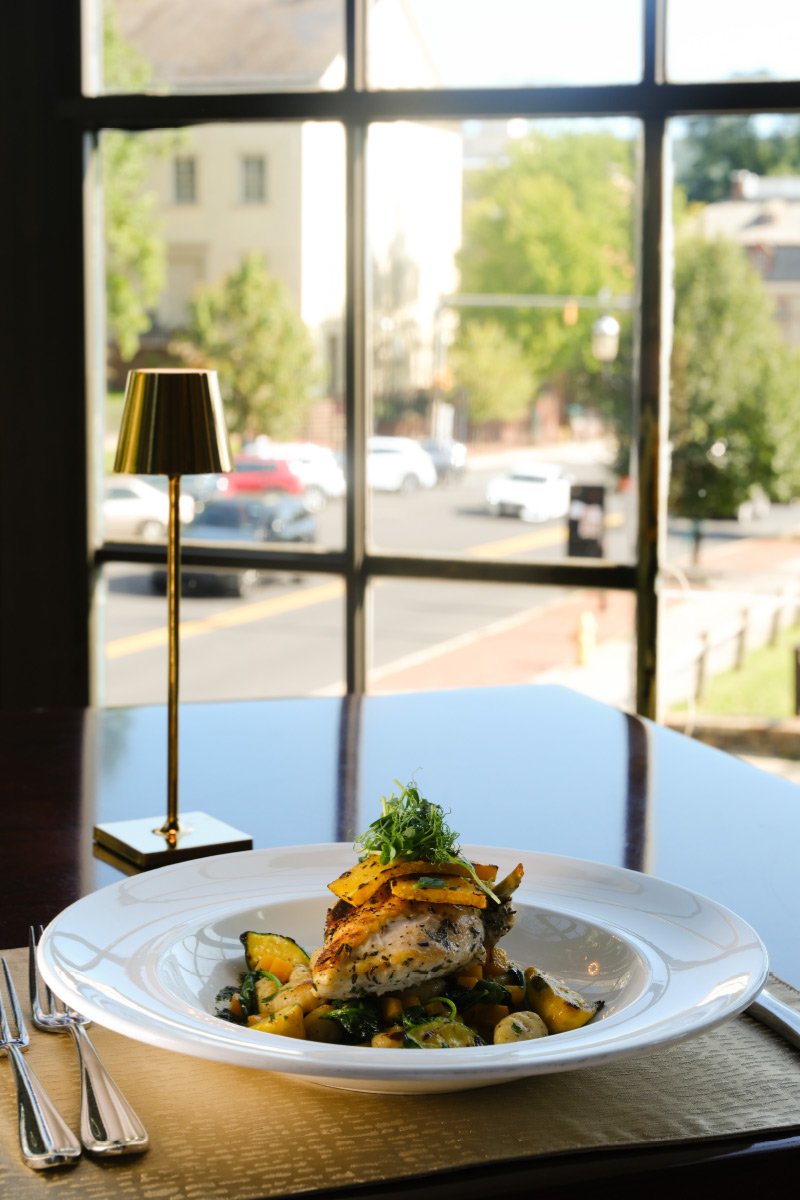The image captures an indoor scene with a focus on a culinary display. The main subject is a white plate set on a light tan table mat atop a gleaming wooden table. The plate contains an artful arrangement of food, starting with a base of assorted green vegetables and what appears to be yellow vegetables. It is topped with a seasoned piece of chicken, adorned with slices of possibly yellow fruit like pineapple, and crowned with a garnish of green leafy stems. Two silver forks are placed to the left of the plate. In the background, through wood-framed glass windows with wooden windowsills, a bustling city street can be seen. Cars navigate the road, some parked, others driving past. Trees line the street, and streetlights add to the urban ambiance. The scene outside is slightly out of focus, drawing attention back to the intricate dish set against the inviting indoor setting. A small golden brass lamp enhances the cozy atmosphere of what seems to be a residential space.